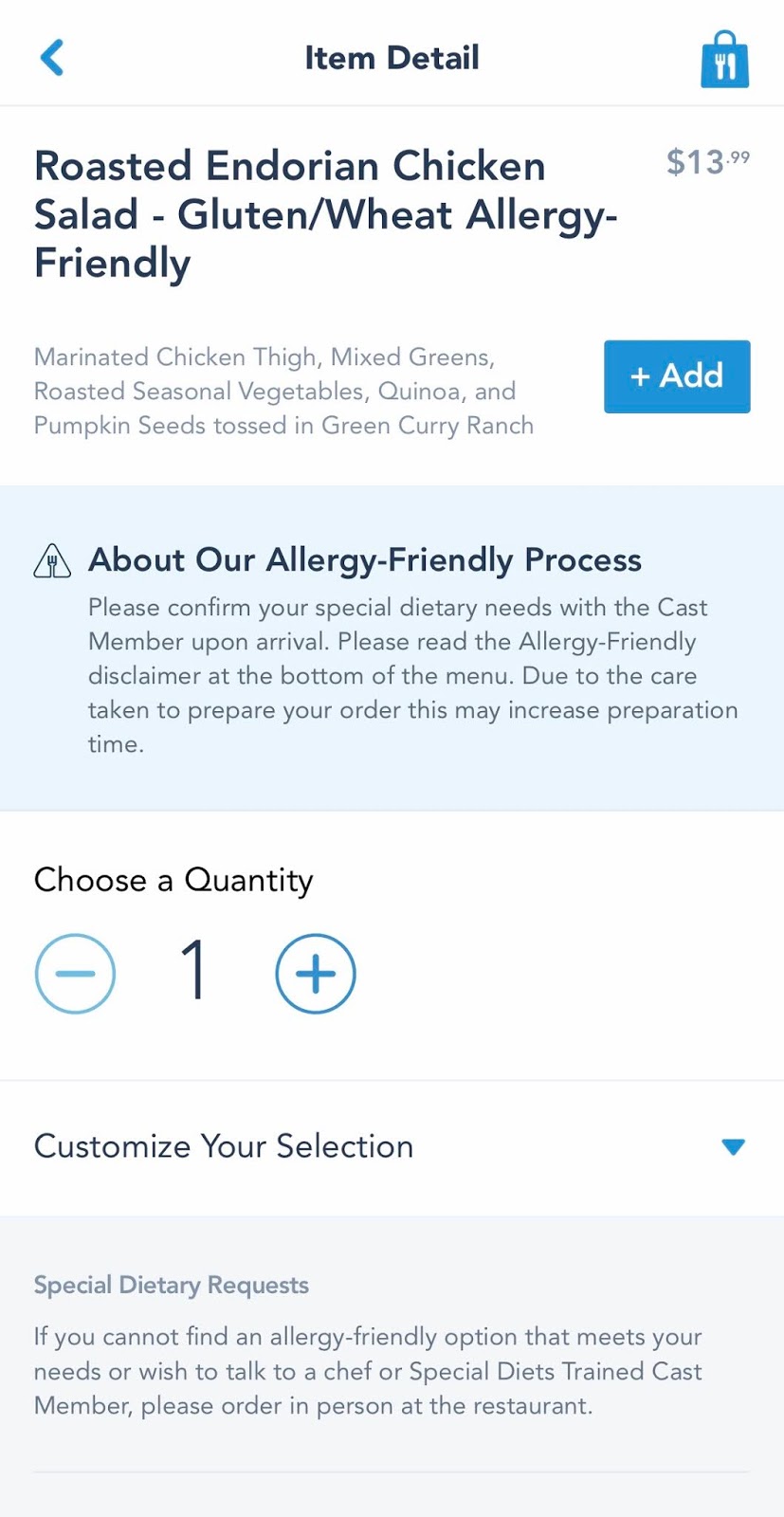The image displays a screenshot of a phone screen showing the details of a specific menu item at the top. The item is a blue bag featuring a fork and knife illustration, labeled "Roasted Endorian Chicken Salad." This dish is highlighted as both gluten and wheat allergy-friendly and is priced at $13.99. 

The description underneath details the salad's contents: marinated chicken thigh, mixed greens, roasted seasonal vegetables, quinoa, and pumpkin seeds, all tossed in a gray curry ranch dressing. 

Additional text advises customers to inform a cast member of any special dietary needs upon arrival and to read the allergy-friendly disclaimer at the bottom of the menu. It also notes that extra care in order preparation may increase preparation time. 

Options to adjust the quantity of the item are provided, currently set at one, with plus and minus buttons available for adjustments.

Customization instructions are included for special dietary requests, suggesting that if a suitable allergy-friendly option isn't found, or if a customer wishes to speak to a chef or special diets-trained cast member, the order should be placed in person at the restaurant. The convenience of ordering ahead of time is also mentioned.